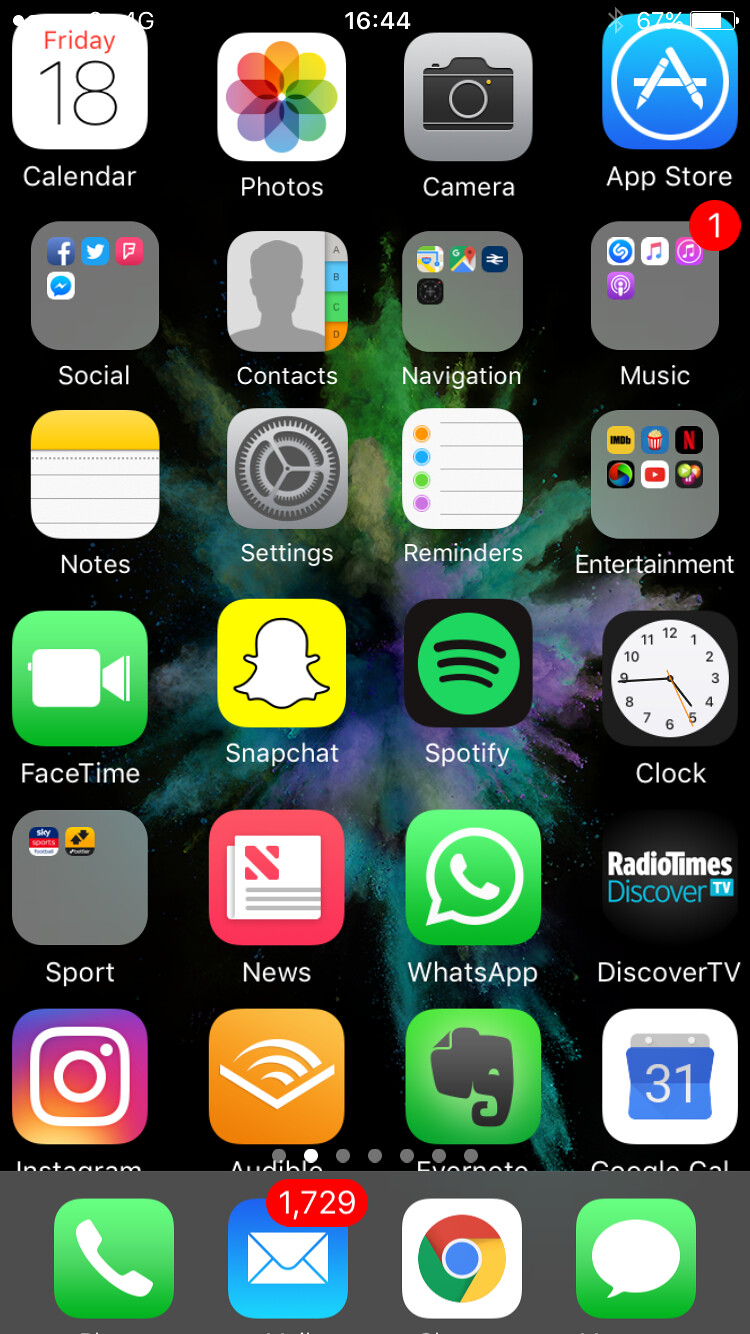Here's a cleaned up and detailed caption for the described image:

---

The image depicts a screenshot of a smartphone home screen, displaying various app icons and details. The time shown on the screen is 16:44 and the battery is at 67%. In the top left corner, the date is indicated as Friday the 18th.

The top row of apps includes:
- **Photos**: Represented by a colorful icon.
- **Camera**: Depicted with a camera icon.
- **App Store**: Marked by a blue icon with styluses forming an "A".
- **Social** Folder: Contains icons for Facebook, Twitter, a red icon possibly for an app with an "F", and Facebook Messenger.

The next row features:
- **Contacts**: Represented by a silhouette of a person's head.
- **Navigation** Folder: Includes two mapping apps, represented by a blue and a black icon.
- **Music** Folder: Contains four music apps, identified by icons of a blue musical note, a rainbow musical note, a purple musical note, and the iHeartRadio logo with a notification badge of 1.

The following row includes:
- **Notes**: Displayed with a notepad icon.
- **Settings**: Shown as a cogwheel icon.
- **Reminders**: Depicted with a checklist icon.
- **Entertainment** Folder: Contains six app icons, including IMDb, a popcorn bucket, Netflix, a circular rainbow swirl, YouTube, and an icon with three globes.

The bottom rows feature:
- **FaceTime**: Displayed with a camera icon.
- **Snapchat**: Represented by a yellow icon.
- **Spotify**: Shown with its recognizable icon.
- **Clock**: Displayed with a clockface icon.

Sequentially, there are:
- **Sports** Folder: Contains two apps within.
- **News**: Depicted in pink and white.
- **WhatsApp**: Shown as a green and white icon.
- **Discover TV**: Includes icons for Discover TV and Radio Times in a black box.
- **Instagram**: Represented by its distinctive icon.
- **Audible**: Displayed as an orange icon.
- **Evernote**: A partially cut-off green icon with an elephant's head.
- **Google Calendar**: Depicted as a white square with the number 31.

At the bottom central part of the screen are the primary navigation icons:
- **Phone**: Green icon for making phone calls.
- **Email**: Displayed with a notification badge indicating 1,729 unread emails.
- **Google Chrome**: Represented by its search icon.
- **Messages**: Green icon with a white speech bubble for text messaging.

---

This detailed caption covers all the elements visible on the smartphone's home screen, providing clear descriptions of each app and its icon.